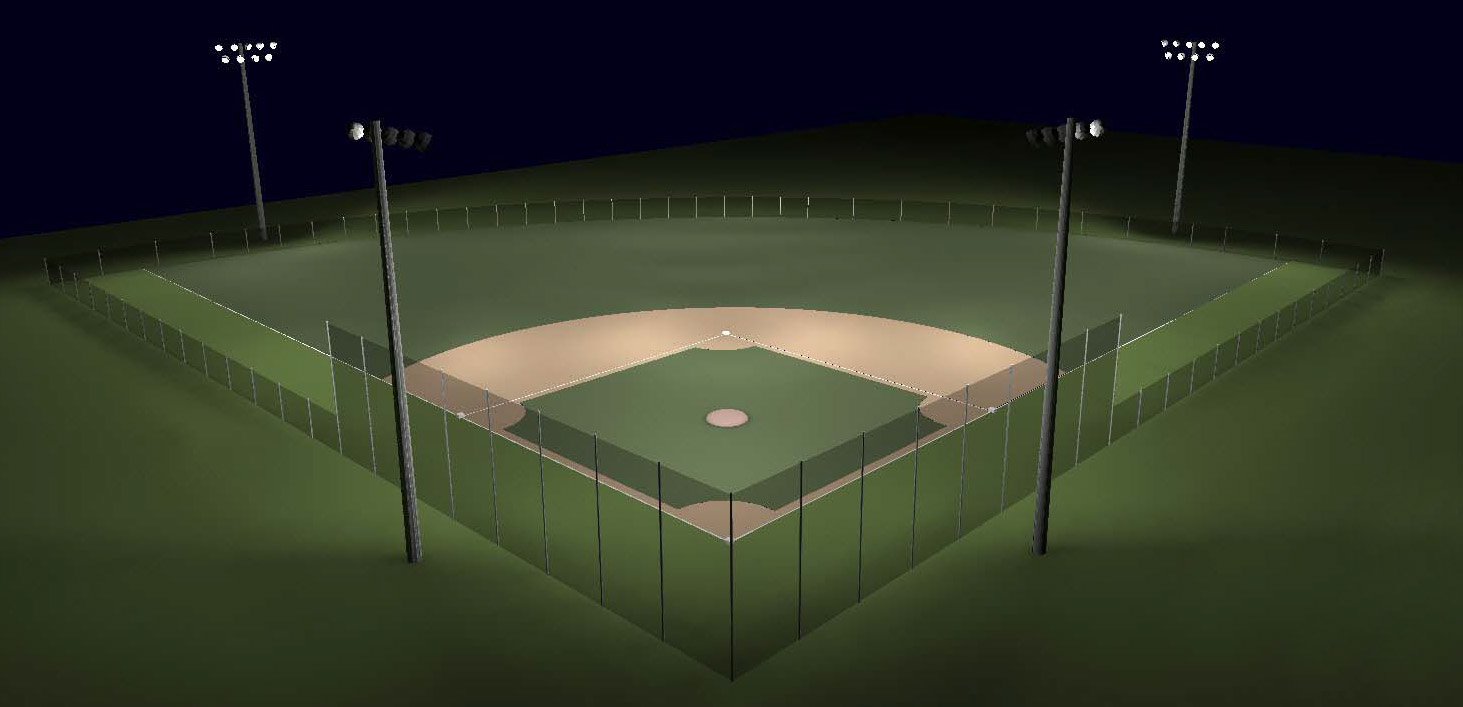The image is a highly detailed and realistic 3D model of a baseball field, appearing at first glance to be a photograph. The field is depicted with a dirt infield and a grass outfield, connected by white chalk lines marking the bases and the pitcher's mound, all bathed in a light that highlights the main center of the scene. Surrounding the field is a comprehensive fencing system: higher fences behind home plate, tapering down from first and third bases to the outfield, and lower fences enclosing the outfield perimeter. The setting is illuminated by four strategically placed light poles—two behind the home plate to the first and third baseline fences, and two beyond the outfield fence—each holding multiple lights. The background of the image is a nearly black, dark blue, giving a stark contrast to the brightly lit field and lending an architectural, almost diagrammatic feel. The scene is devoid of players, spectators, or text, focusing purely on the structural details of the empty baseball diamond.